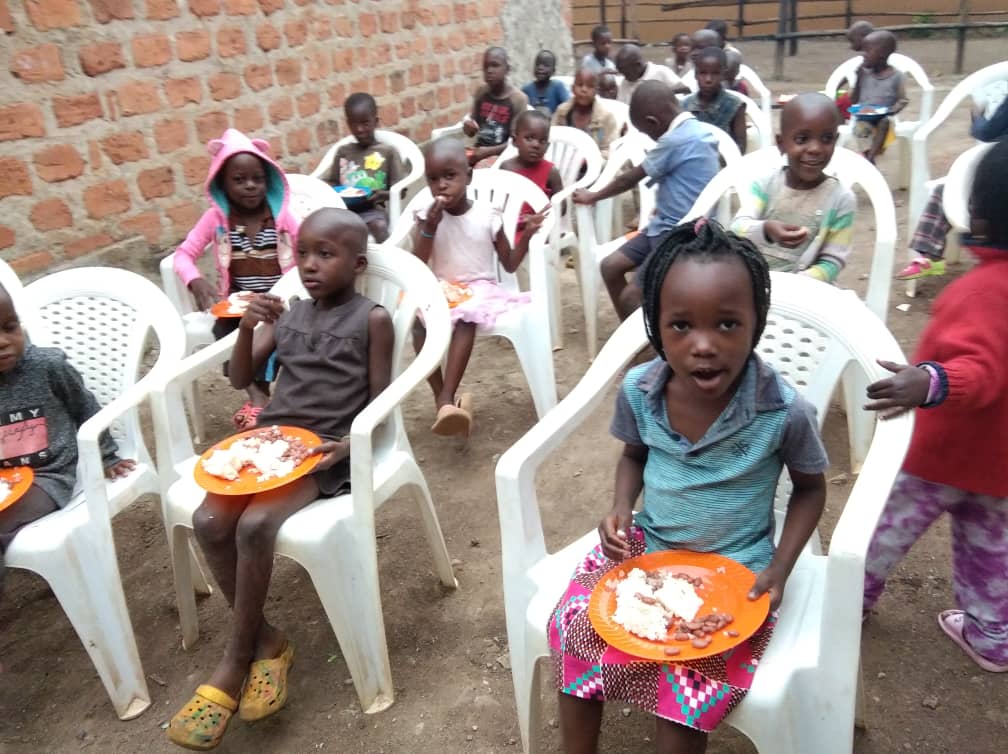The image depicts a large group of children seated in plastic lawn chairs arranged in rows. Most of these children appear to be of African or African American descent. They are having a meal served on orange plastic plates, though no utensils are visible. The children are largely focused on eating, except for one who is walking between the rows heading toward a friend, and a few others who seem relaxed and laid-back. The food on their plates consists of a white substance resembling grits, and some beans, giving the impression of a simple meal. In the background, metal fencing and rails are visible, along with brick walls to the left, suggesting that this could be an outdoor school setting where the children are having their lunch.